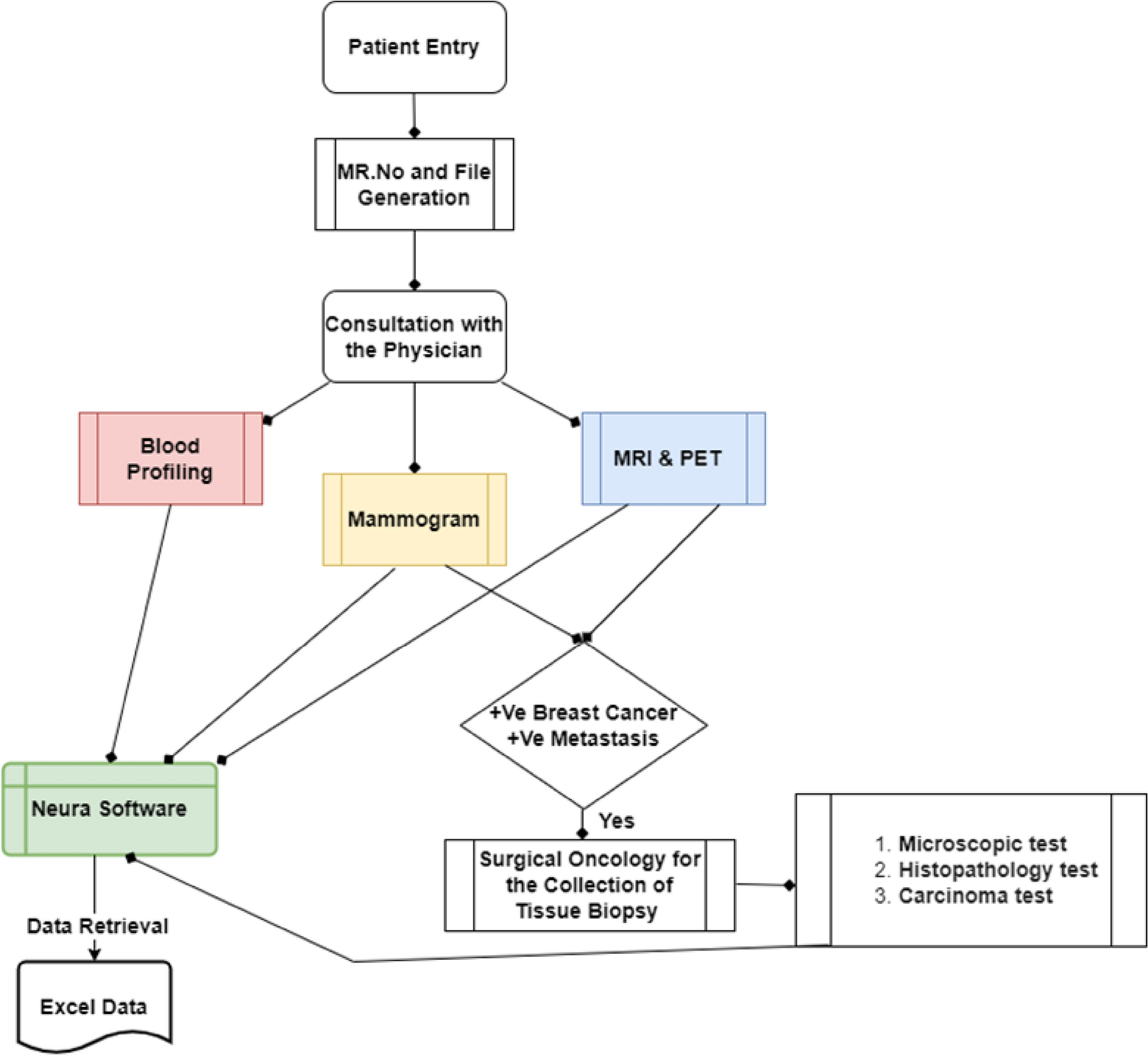The image showcases a detailed medical flowchart with a white background and several color-coded rectangles indicating various steps and processes in a patient's medical evaluation and treatment. At the top of the flowchart, enclosed within a black rectangle, the process initiates at "Patient Entry," followed by "MR Number and File Generation." A line extends downward to "Consultation with the Physician," from which three branches emerge. 

The left branch leads to a red rectangle labeled "Blood Profiling;" the middle branch, in yellow, indicates "Mammogram;" and the right branch, in blue, points to "MRI and PET." Each of these branches converges into a green rectangle marked "Neuro Software," which subsequently leads to "Data Retrieval" and "Excel Data."

Concurrently, the middle "Mammogram" and right "MRI and PET" branches also channel towards a diamond-shaped box labeled "Positive Breast Cancer, Positive Metastasis." This leads into "Surgical Oncology for Collection of Tissue Biopsy," followed by three subsequent tests: "Microscopic Test," "Histopathology Test," and "Carcinoma Test." 

The flowchart effectively outlines the sequential steps and decision points in the medical diagnosis and treatment of breast cancer, incorporating various diagnostic techniques and follow-up procedures.